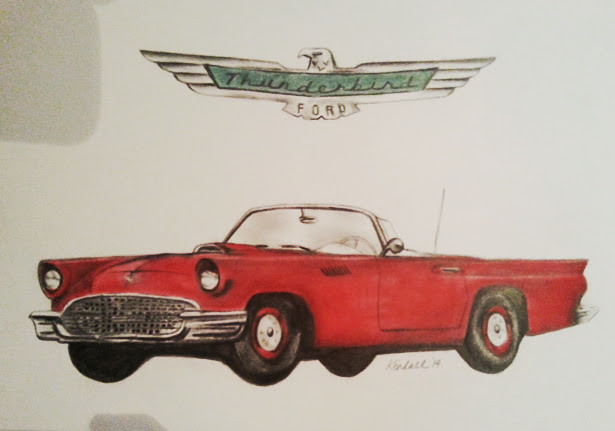The image depicts a detailed sketch of a classic vintage Ford Thunderbird convertible, prominently colored in bright red. The car is illustrated with the top open, showcasing its timeless design reminiscent of the 1950s era. The front of the Thunderbird features a silver chrome grille and bumper, adding a touch of elegance. The wheels are accented with a red trimming around the circumference. Above the car is the iconic Thunderbird logo, featuring an eagle with stylized long, narrow wings looking to the left. The logo includes the word "Thunderbird" in a script font set against a green background, and the Ford logo beneath it. The entire composition has a notable shadow, suggesting the artwork might be attached to a wall or that there's an external object casting shadows. At the bottom of the sketch, there's a signature reading "Kendall H.," suggesting the artist's attribution.